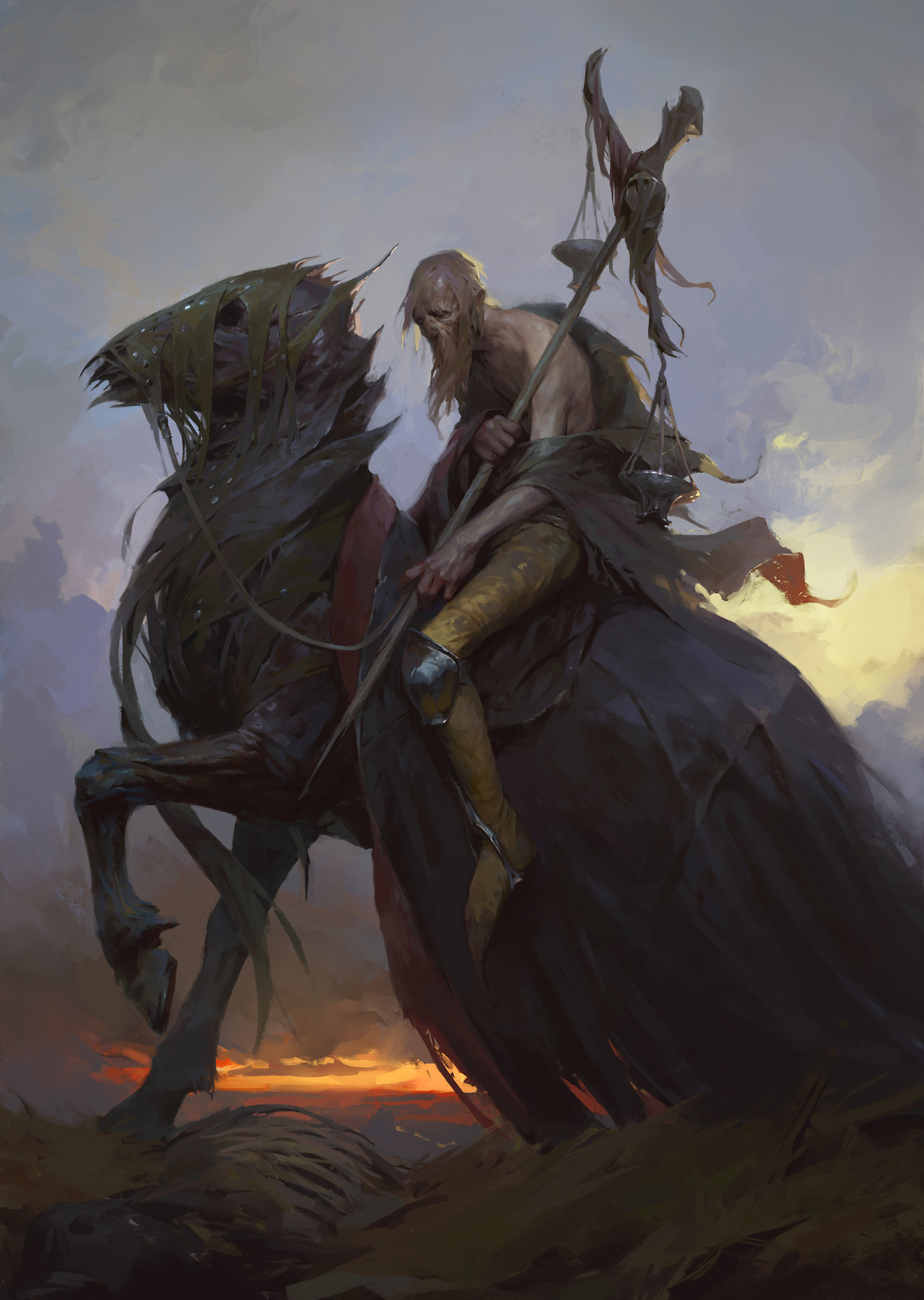This eerie image, illustrated in dark, ominous tones, depicts an apocalyptic scene with a stormy, gray sky dominating the background. The landscape is accentuated by deep brown and green long grass, appearing muddy and desolate. Above this desolate terrain stands a grotesque horse-like figure adorned with long grass or seaweed entwined in its mane. The horse's head and neck are distorted with spiky protrusions, and it is draped in black fabric that obscures its back legs, adding to its statue-like, unnatural appearance.

Atop this ghastly steed sits a man, emaciated and shirtless, with pallid skin and a haggard, bearded face, evoking the image of someone who has endured harsh, prolonged hardships. The rider is slumped slightly forward, clutching an elongated weapon resembling a dagger or staff that features a prominent metal part near its top, with tattered fabric dangling from it. His attire is equally worn, with tattered robes and a knee pad visible on one leg, revealing a yellowish hue on the exposed part of his limb.

The setting enhances the macabre scene, with an orange spot resembling fire at the bottom, suggesting a burning landscape, and a small yellow patch in the otherwise bleak sky towards the middle right. The entire composition, from the haunting figures to the apocalyptic background, combines to create a chilling, dark fantasy tableau.